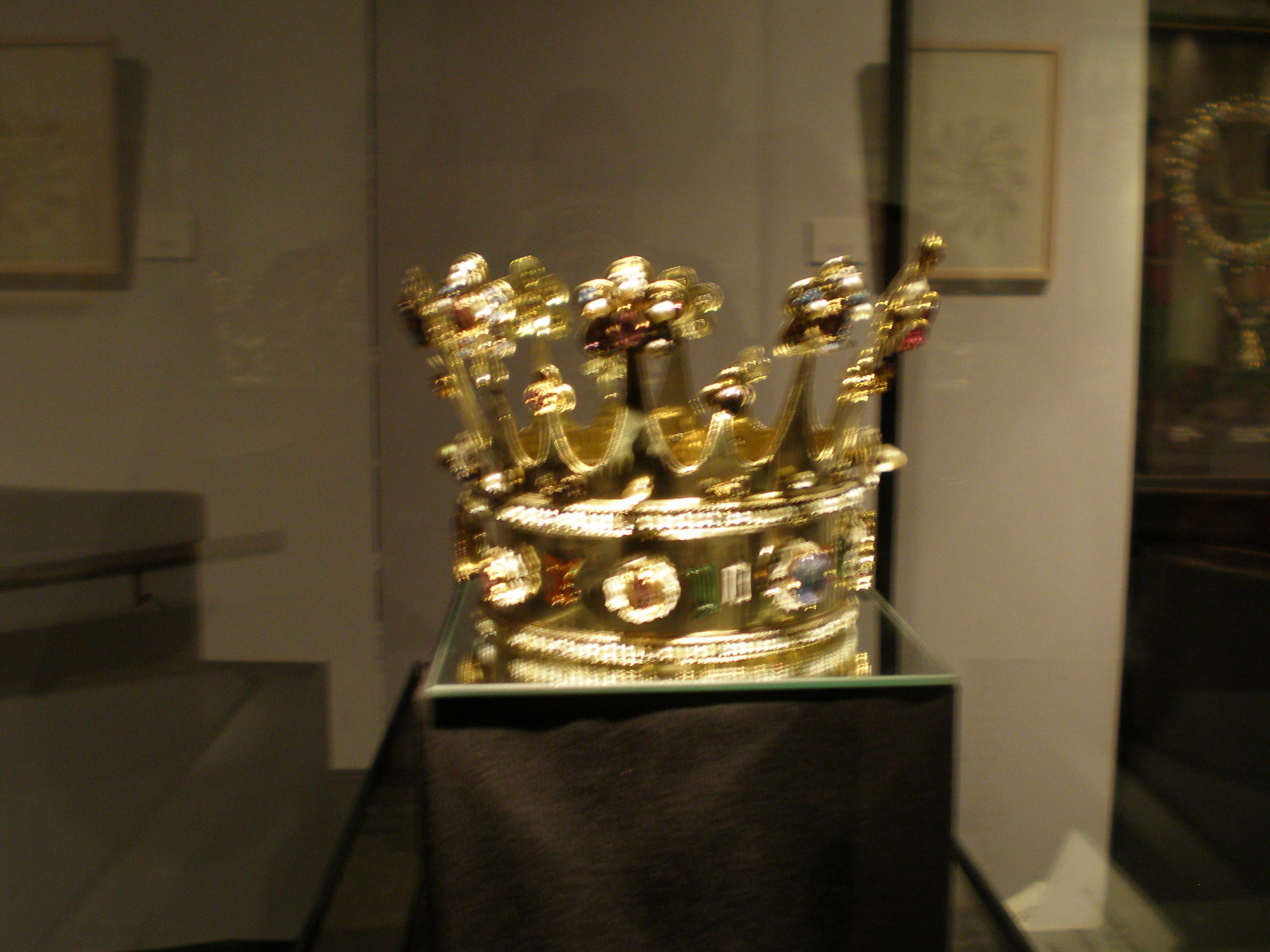The photograph depicts a highly ornate, gold crown encased in a glass display within what appears to be a museum setting. Despite the image being blurred, perhaps due to a slow shutter speed or camera movement, several details are visible. The crown, encrusted with an array of colorful jewels including rubies, emeralds, and sapphires, sits atop a raised platform draped in wrinkled black cloth. This platform features a mirror-like top surface, reflecting the crown's intricate design. The crown's circular base is adorned with jewels, and its familiar undulating U-shaped peaks rise to form pointed triangles, each capped with jewel-encrusted leaf motifs. Surrounding the central display are museum walls showcasing additional artworks and memorabilia. The glass case housing the crown reflects ambient elements, including other exhibits, stairs, and the faint images of two individuals taking the photograph. The museum appears dimly lit, adding to the reflective quality of the glass case. Visible in the reflections are both the photographer and a second person, contributing to the layered complexity of the scene.